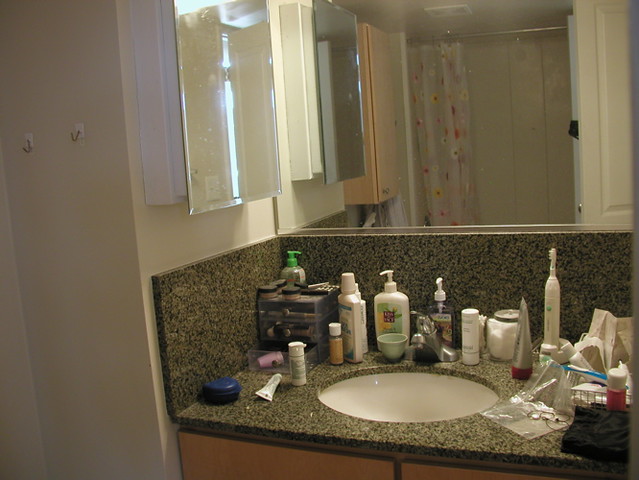This photograph captures the detailed interior of a washroom with pristine white walls. Dominating the foreground is a sleek black countertop, speckled with lighter dots, which seamlessly extends up onto the wall behind. At the center of the countertop lies a gleaming white sink, supported by brown cupboard doors underneath. Above the countertop is a prominent mirror, reflecting various elements of the bathroom. The reflection reveals a white door, a neatly organized shower area with a white and pink polka-dotted curtain, and a cabinet door.

The countertop is laden with various items, contributing to a lived-in yet organized ambiance. On the far left sits a distinctive blue circular object next to a white tube. In the corner, an elegant box-like container for storage is visible. Adjacent to it is a white bottle equipped with a pump, followed by a clear bottle with a similar pump top. A few more tubes are scattered nearby, along with a white electric toothbrush standing upright. To the right of the counter, a small pile of papers and sundries can be seen, partially covered by a black cloth, adding a touch of realism to the scene.